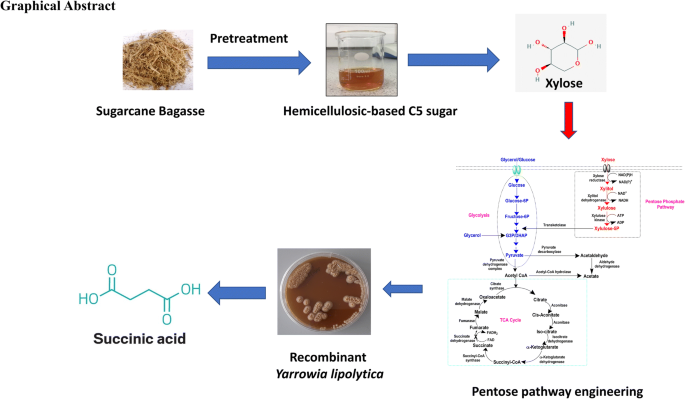The graphical chart on an all-white background, titled "Graphical Abstract," begins at the top left with black text reading "sugarcane bagasse" alongside an image depicting a pile of brown plant material. A blue arrow labeled "pretreatment" points to the right towards a glass jar marked "hemicellulosic-based C5 sugar," containing a brown liquid. Further to the right, another blue arrow points to a chemical compound chart segmented into various sections. Below this, a red downward arrow leads to a larger chart detailing components labeled "Pentose Pathway Engineering." A blue leftward arrow labeled "recombinant Yarrowia lipolytica" points to an image of a cup filled with a brown liquid, resembling hot cocoa with lighter brown particles floating in it. Another blue leftward arrow extends towards more chemical notations, including HO, O, OH, indicating succinic acid on the left.